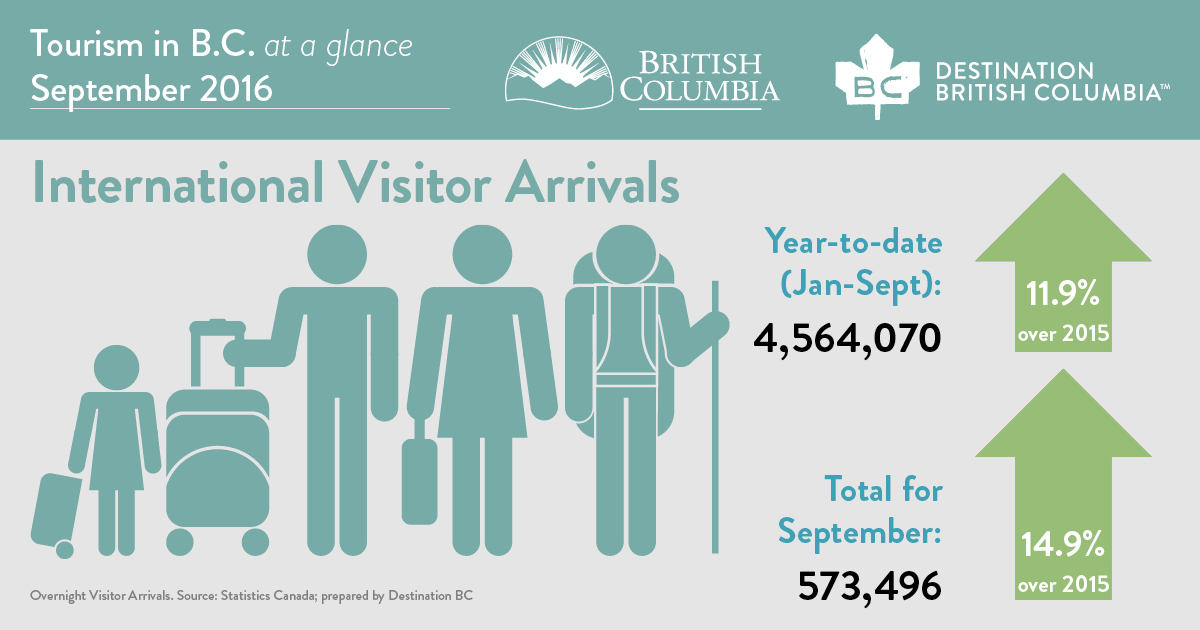This image is a horizontally aligned rectangular graphic detailing international visitor arrivals for tourism in British Columbia as of September 2016. The top quarter of the image features a teal banner with white text that reads "Tourism in BC at a Glance," followed by "September 2016." To the left, there's the British Columbia logo, including a sun and mountain outline, adjacent to a white leaf with "BC" inside it. The phrase "Destination British Columbia" is also displayed in white text.

Beneath this banner, the remaining three-quarters of the image has a light gray background. On the left side, it says "International Visitor Arrivals" in gray print. Alongside this text are four teal stick figures: an adult with a suitcase, a child with a smaller suitcase, another adult with a briefcase, and a third adult with a backpack. There is a vertical line separating this section from the right side information.

On the right, blue text states "Year to Date Jan-September," followed by the number "4,564,070" in black. To the right of this, a blue up-arrow indicates an 11.9% increase over 2015. Below, "Total for September" is written in blue, with "573,496" in black below it. A green up-arrow alongside shows a 14.9% increase over 2015.